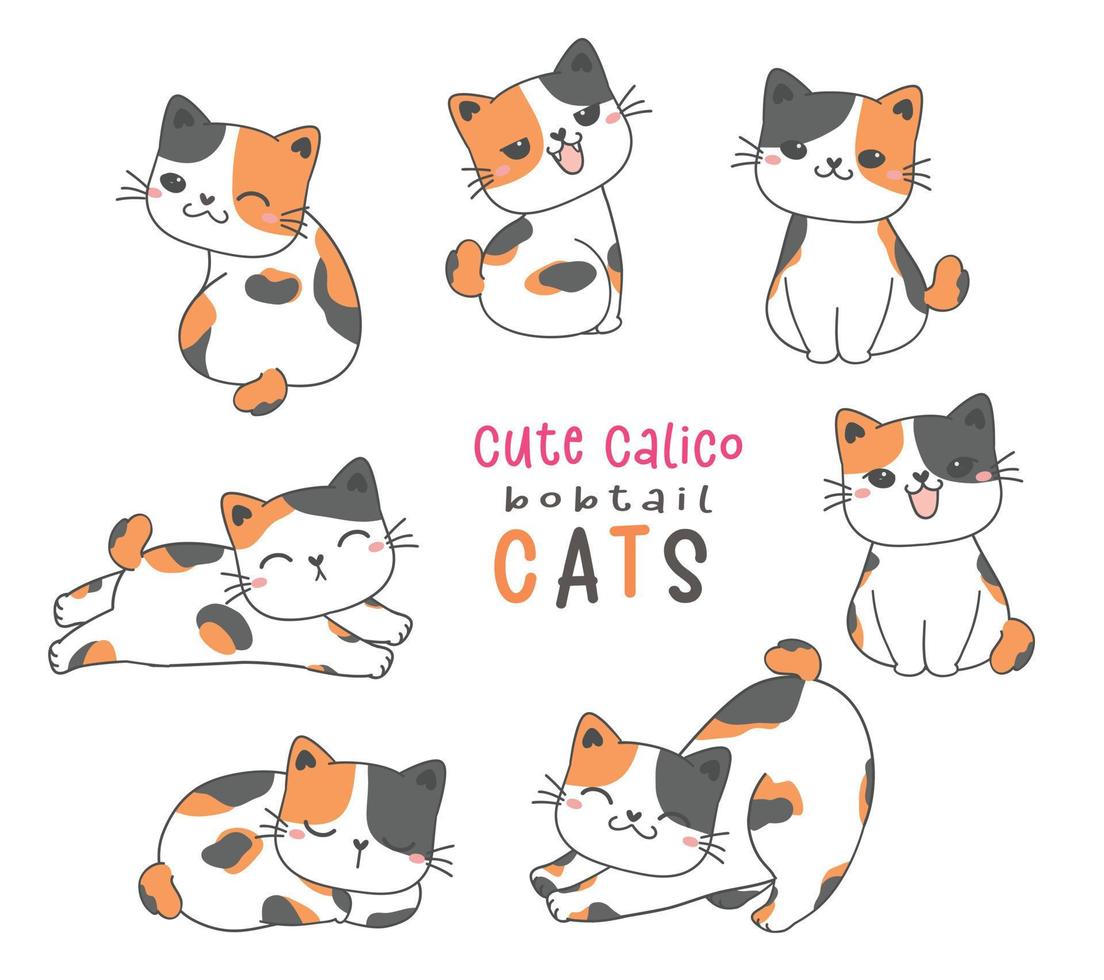This detailed illustration features an adorable collection of seven kawaii-style calico bobtail cats encircling the central text that reads "Cute Calico Bobtail Cats." The text is visually appealing with "Cute Calico" in a pinkish-red color, "Bobtail" in black, and "Cats" in alternating orange and black. Each of the seven calico cats showcases a unique personality and emotion. 

In the top left, there's a cat winking back at the viewer while turning its head. Adjacent to it on the right is a cat with a wide, smug-looking smile. Further right, another cat sits with a content, closed-mouth smile, a hint of blush beneath its eyes. A cat on the top right appears to be smiling happily.

On the bottom right, one cat is stretching with its bum up and eyes closed, suggesting contentment. The bottom left features a cat napping, curled into a cozy ball, while the final cat on the left side is also napping but stretched out with its forelegs extended in front and hind legs behind.

Each cat is a charming blend of orange, black, and white splotches, representing the quintessential calico patterns, and together they create a scene full of warmth and playful demeanor.